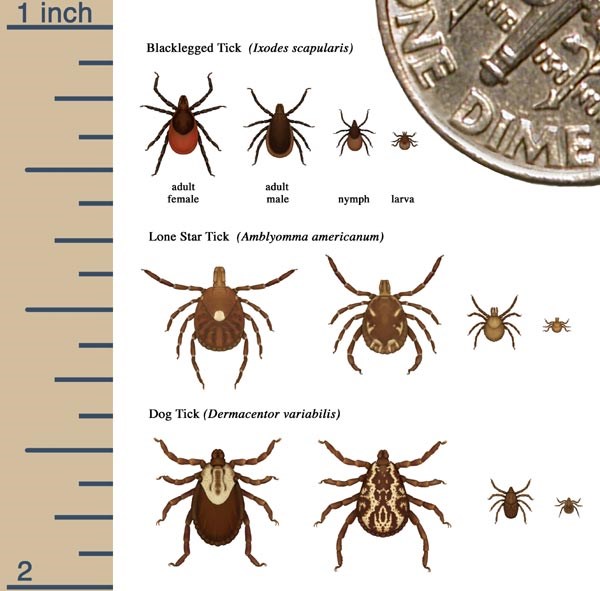The image is an infographic illustrating three types of ticks, each detailed with their scientific names and stages of development. On the left side, a ruler scaling from one inch to two inches serves as a size reference. The ticks presented are: the Black-Legged Tick (Ixodus scapularis), which is shown in its adult female, adult male, nymph, and larva stages; the Lone Star Tick (Amblyomma americanum), recognizable by a distinctive white dot on its back; and the Dog Tick (Dermacentor variabilis). All ticks are depicted as various shades of brown. To further provide a sense of scale, a United States dime is shown in the upper right corner of the image.